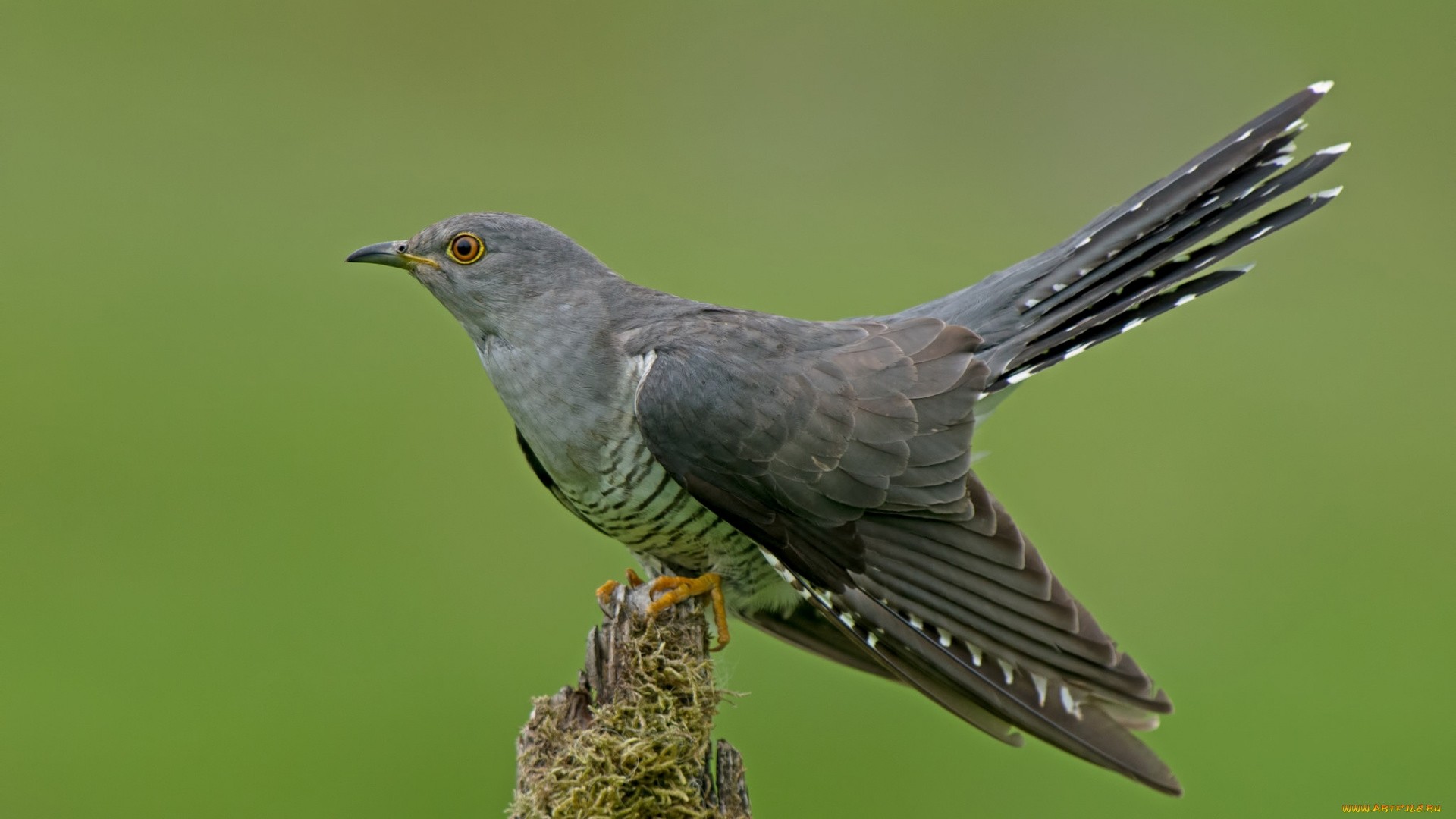The image features a nature scene with a light green or sage background, which is medium green in color, possibly blurred or solid. The focal point is a bird that occupies the center of the image, perched on a piece of moss-covered wood. The bird has distinctive features, including medium gray head and neck, with white and black striped underbelly. Its wings are a mix of black, chocolate, and gray, accented with white details. The bird also has striking copper-colored eyes with black pupils, a black beak, and orange talons. The image lacks any additional objects or text, focusing solely on the detailed, close-up view of the bird.